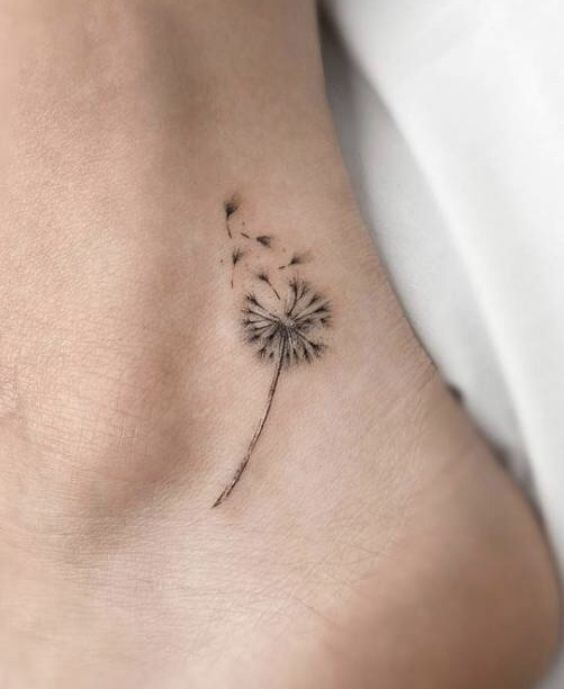In this close-up image, we're looking at the left side of a person's light-skinned heel adorned with a detailed black ink dandelion tattoo. The tattoo is located just above the heel, proximate to the Achilles tendon, and depicts a dandelion with some of its seeds gracefully blowing away in the wind. The delicate stem of the dandelion angles towards the bottom left, while the blossom with its dispersing seeds points towards the top right. The person's foot rests on a white blanket that occupies the remainder of the image, providing a soft, contrasting background to the intricate design. The subtle detailing of the tattoo, combined with the natural skin tone and the minimalistic setting, draws attention to the delicate charm of the wind-swept dandelion.